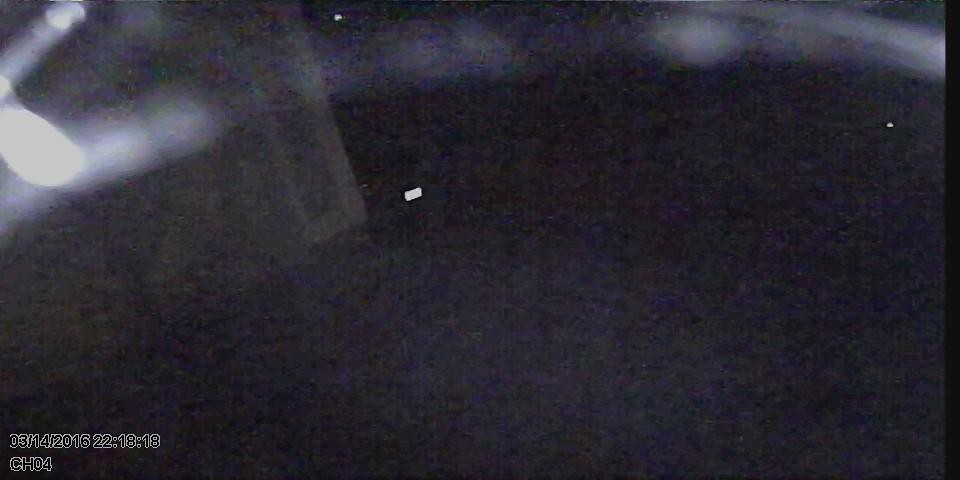The image appears to be a blurry frame, likely captured from an outdoor security camera or doorbell cam, possibly mounted at an elevated position such as a garage. The central focus of the image is largely indistinct, marked predominantly by a dark, black, shiny area, which might be an object reflecting some light. The most discernible element is a small, white license plate centered in the image, without any visible text due to the heavy blur. Light reflections are evident, particularly in the upper left, where a glare or reflection catches the eye. The bottom left corner of the image features a timestamp, reading "03/14/2016 22:18:18," and the text "CH04" below it, indicating this is the fourth channel of the security system. Overall, the image's clarity is compromised, making it difficult to extract any more specific details.